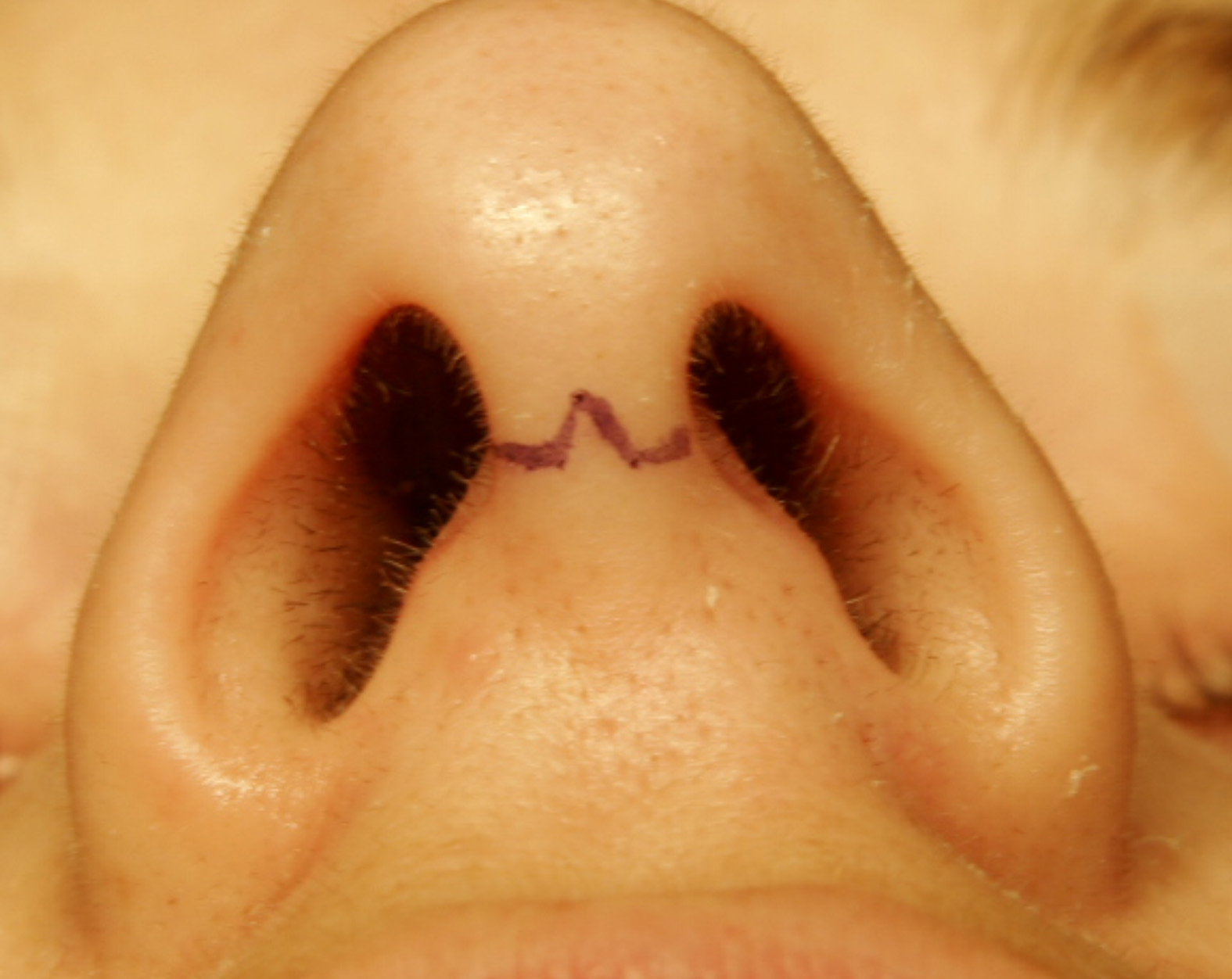The image is a close-up photograph of the underside of a person's nose, prominently displaying both nostrils at either side. The composition centers around the nose, where there is an intriguing pen marking. This marking starts at the tip of the nose and forms an upside-down V shape, with lines extending horizontally outwards from the apex of the V towards each nostril. The nose hair is visible within the nostrils, which is a normal detail. The surrounding skin appears in shades of beige, light brown, and tan, with the face in the background slightly blurred. This unusual marking on the nose raises questions about its purpose, potentially suggesting either a prelude to plastic surgery or a playful, albeit cryptic, joke.